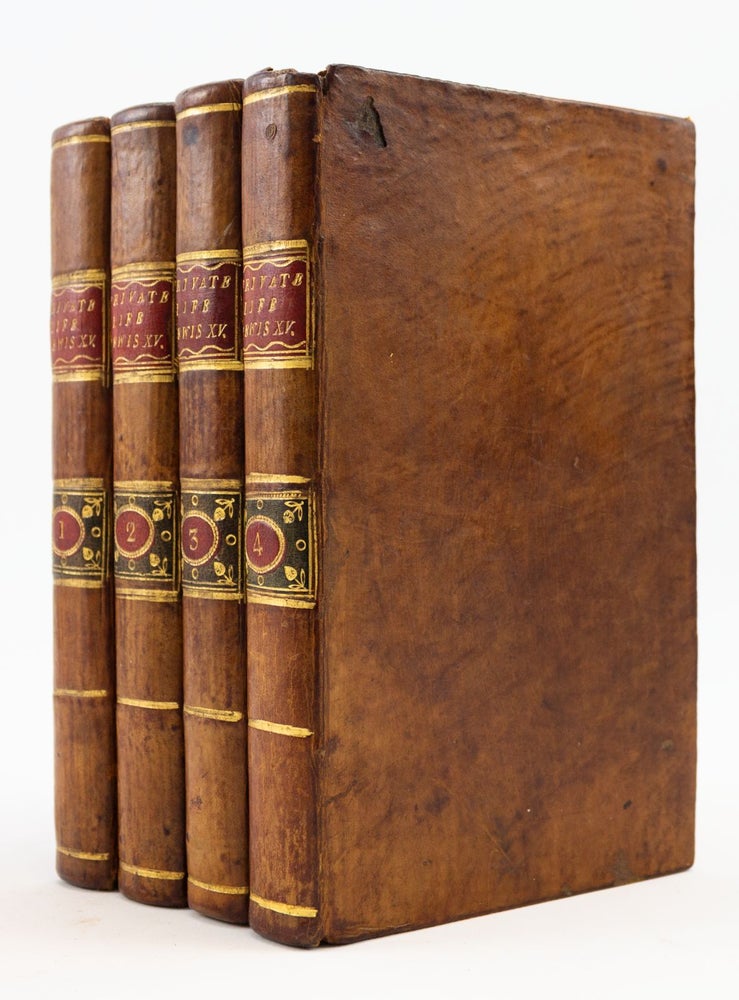This color image captures four vintage, leather-bound books, lined up tightly against a white background. The books, which appear well-worn with numerous dings and age marks, suggest they are several decades old, possibly encyclopedias. Their spines feature a rich combination of brown leather, gold stripes, and red accents. Each volume is labeled consecutively from 1 to 4, with the numbers encased in gold-trimmed circles that are maroon inside. Decorative gold designs, including a rose pattern, adorn the spine against a black background. Although some text is legible, indicating "The Private Life of [unidentifiable word]," the majority of the print details are obscured, hinting at a wealth of hidden knowledge within their pages. This nostalgic image evokes memories of a time when such books were essential for study and discovery in libraries.